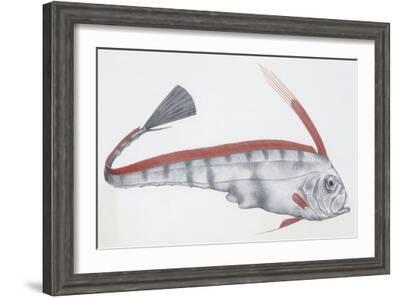This small image depicts a framed drawing or painting of a unique fish, set against a completely white background. The piece is mounted within a wide rectangular dark gray wooden frame, which casts a slight shadow behind it in the bottom left corner. The left side of the frame appears closer than the right, indicating a slight tilt.

Inside the main frame, a white cardboard mat surrounds the fish artwork. The fish faces right, characterized by a long gray body with dark gray stripes that widens near the head and curls back, creating a recognizable shape. The fish features a distinct red fin along its back and another enigmatic red, pointy appendage jutting from the top of its head. Additional small red fins can be seen at the bottom of the fish. Above its head, a diagonally vertical red stripe extends upward, perhaps elaborating on the intricate detailing along its form. The tail, which fans out expansively, resembles the bristles of a paintbrush or the spread of a traditional fan, further accentuating the artwork's detail and fluidity.